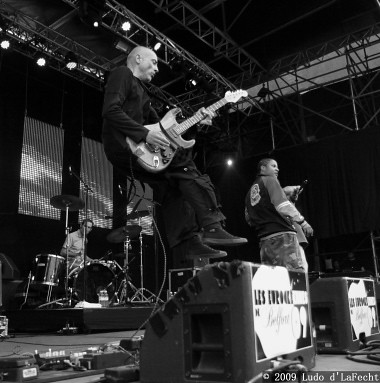In this detailed black-and-white image, we see a live band performance captured from the stage. The scene is set in an industrial-like venue with a hard surface ground, possibly concrete, and various mechanical setups, including spotlights and the stage frame. At the center of the image is a bald guitarist with short hair, seated on a tall stool, his feet dangling over the speaker system, and dressed entirely in black, including black Converse shoes. He is playing an electric guitar. Behind him, a drummer is positioned, playing a black drum set. To the right, a singer stands, clad in a jacket with long sleeves and camo cargo pants. The setting is adorned with various lighting fixtures from the ceiling and scattered around are amplifiers. The scene exudes a mix of industrial and musical ambiance, and in the bottom right corner, the image bears the text "Copyright 2009, Ludo De La Fecte."